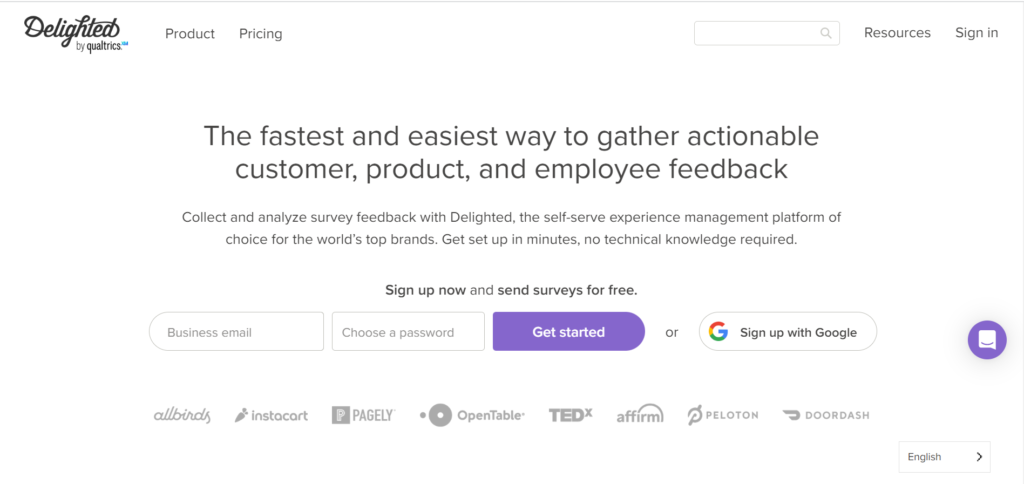This is a home page of a website with a predominantly white background. Along the top, there's a thin gray border. Positioned in the top left corner, the word "Delighted" is prominently displayed in bold, cursive black font. Directly beneath the "Delighted" text, in smaller black letters, it reads "by Quality Matrix".

To the right of "Delighted", the navigation bar includes the following options: "Product" and "Pricing" on the left, followed by "Resources", and finally "Sign In" on the far right. Below this navigation bar, about two inches down in the center of the page, there's a prominent rectangular search bar.

Centrally positioned in large black letters is the tagline: "The fastest and easiest way to gather actionable customer, product, and employee feedback." Following this tagline, two lines briefly describe the company's services. 

There is a call-to-action button centrally located that states: "Sign up now and send surveys for free". Below this, slightly to the left, there is a rectangular-shaped input box for "Business Email" with a rounded left side. To its left is another input box for "Choose a password". Adjacent to these input boxes, there's a purple button with white text that reads "Get Started".

Alternatively, users can "Sign up with Google" using the white tab featuring the Google "G" icon on the left. Below these sign-up options, there's a purple circle with a white square inside it.

At the bottom left-hand corner of the page are logos of companies that support the platform. They include Allbirds, Instacart, Paisley, OpenTable, TED, Affirm, Peloton, and DoorDash, each accompanied by their respective icons. Finally, in the bottom right corner, in very small black lettering, it says "English".